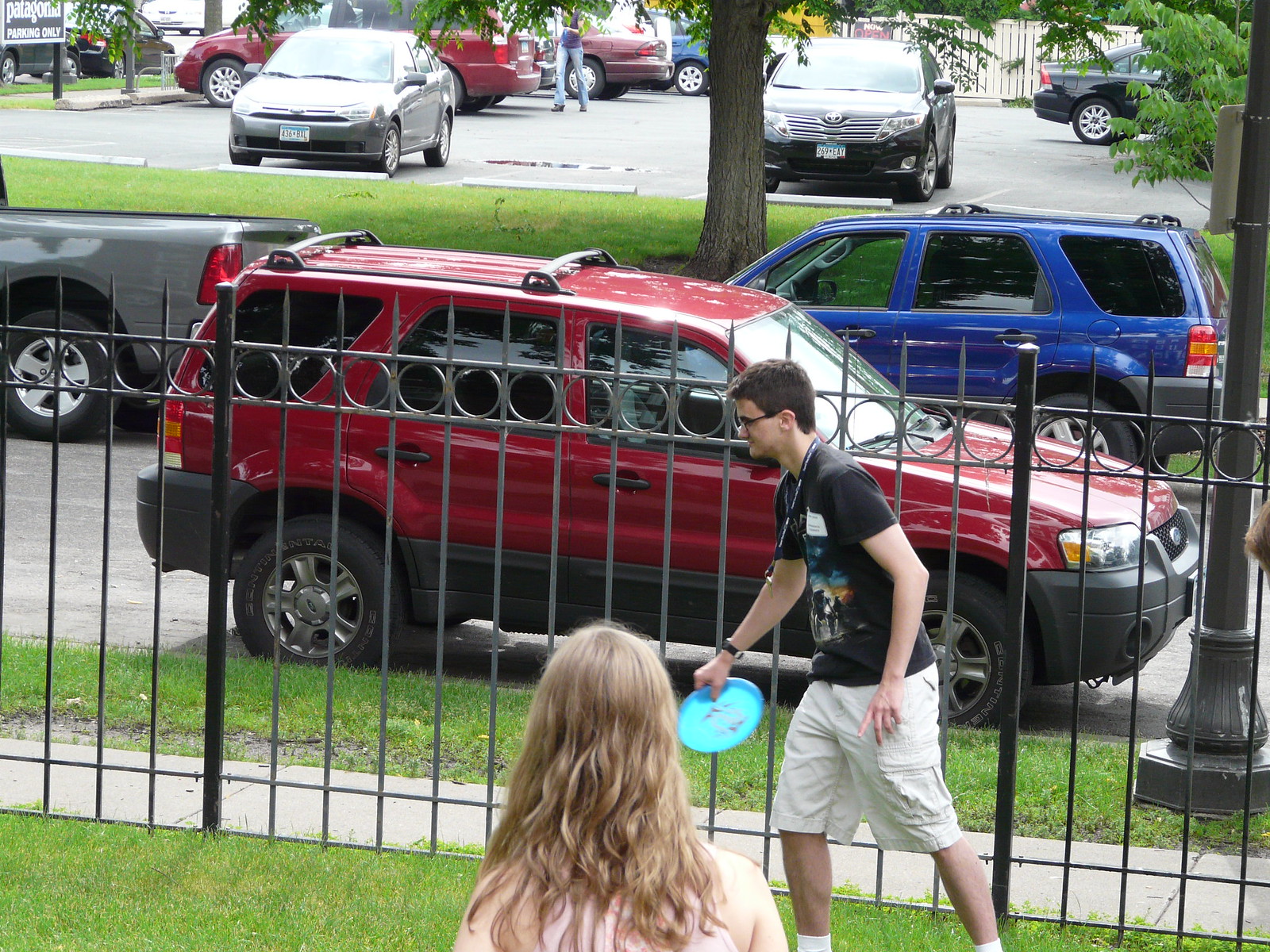This image captures an outdoor scene in a park on an overcast day. In the foreground, a young girl with long, wavy blonde hair is seen from behind, her shoulders visible in a sleeveless top. Just ahead of her is a young boy characterized by his black t-shirt, khaki cargo shorts, glasses, and a lanyard around his neck. He holds a turquoise-blue frisbee in his right hand, as if ready to throw it. The grassy area they occupy is enclosed by a tall iron fence with vertical and horizontal bars adorned by circular motifs.

Beyond the fence, there is a narrow strip of grass followed by a sidewalk. A black metal light post stands on this strip. Parked along the adjacent street, a red SUV faces to the right while a blue SUV faces left across the street. The far left of the photograph reveals the back end of a gray pickup truck. Further back, a larger patch of grass with scattered trees separates the street from a slightly elevated parking lot filled with various cars. The parking lot, which appears to belong to a Patagonia store, features multiple vehicles aligned in different directions, framed by more trees and plants in the distance. The overall setting evokes a tranquil, neighborhood atmosphere with a mix of everyday activity and play.